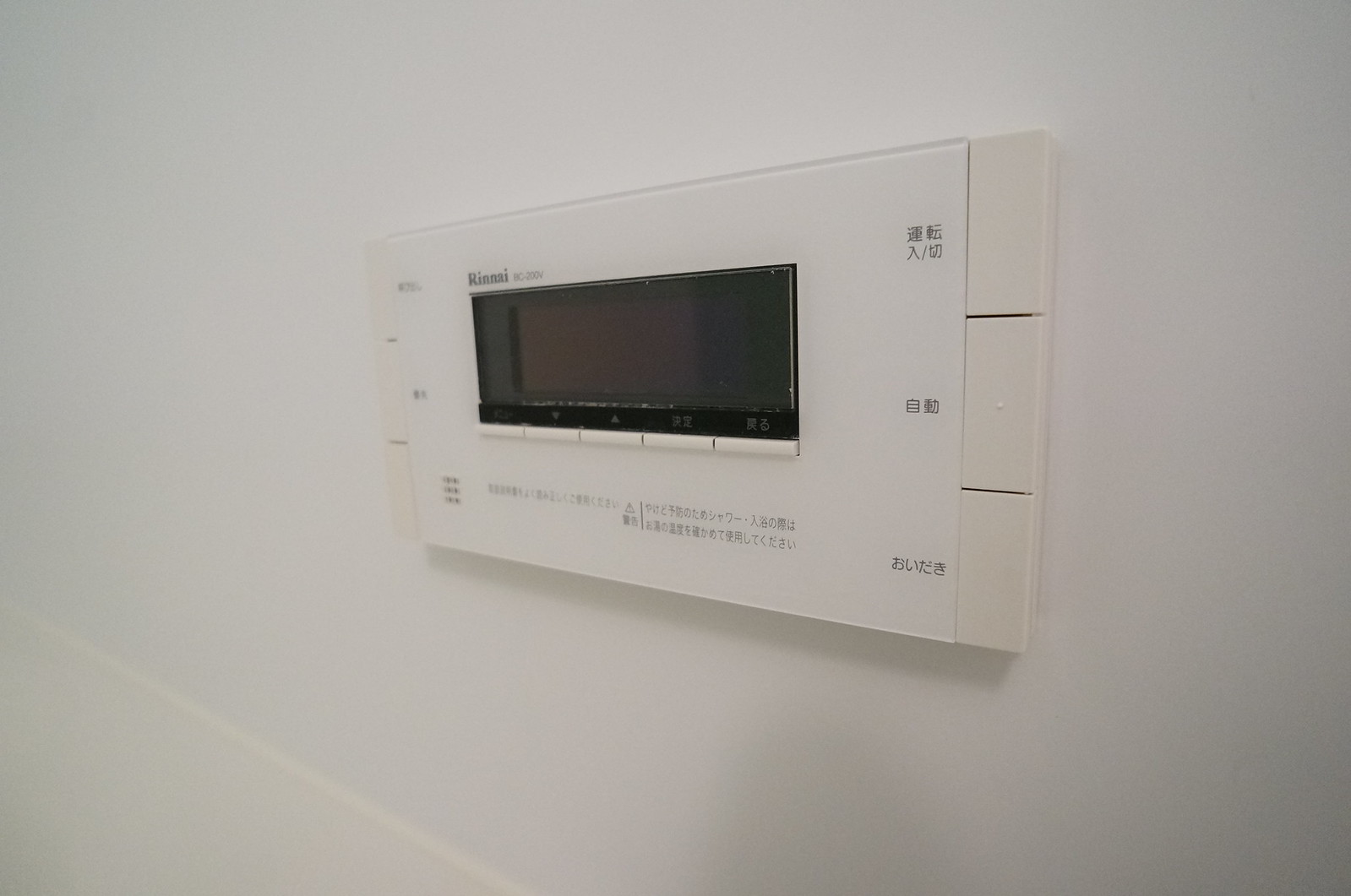The image depicts a minimalist white wall adorned with a sleek, rectangular electronic device, resembling a wall thermostat. This device features a glossy, black glass face that mirrors the rectangular shape of its plastic body, providing a sharp contrast against the white wall. The glass face displays various data and is adorned with characters in what appears to be an East Asian language, possibly Japanese or Chinese, labeling different functions and settings. Prominently positioned at the top of the glass face is the brand name "RINNAI" spelled out in capital letters. The other characters remain undecipherable due to their foreign script. The overall design is clean and modern, highlighting the device's sophisticated functionality and international origin.